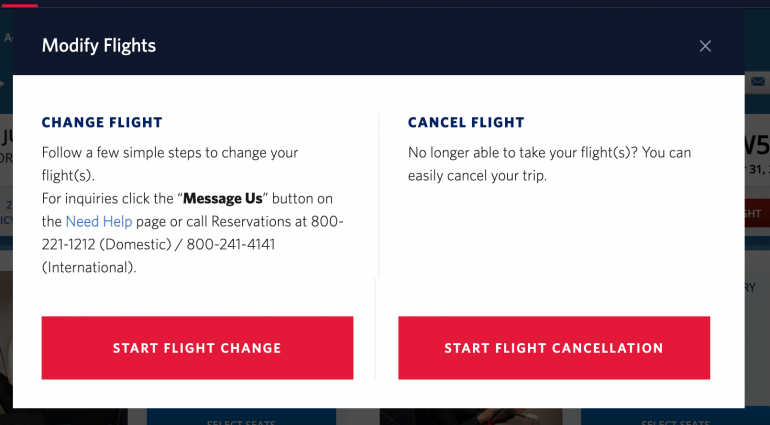The image appears to be from an airline's website, focusing on flight modifications. The section has a dark background with contrasting white text that reads "Modify Flights." On the top-right corner, there is a light gray "X," indicating an option to close the window.

The content is divided into two sections by a vertical light gray line. The left section deals with changing flights. The headline "Change Flight" is in blue text. Below it, in black text, it instructs: "Follow a few simple steps to change your flights. For inquiries, click the 'Need Help' link or call reservations at 800-221-1212 (domestic) or 800-241-4141 (international)." The "Need Help" link is also in blue, likely clickable for user assistance. Beneath these instructions, there is a prominent red rectangle with white text, "Start Flight Change."

The right section addresses flight cancellations. The headline "Cancel Flight" is in blue text. The accompanying black text states: "No longer able to take your flight? You can easily cancel your trip." Similar to the left section, there is a large red rectangle with white text that reads "Start Flight Cancellation."